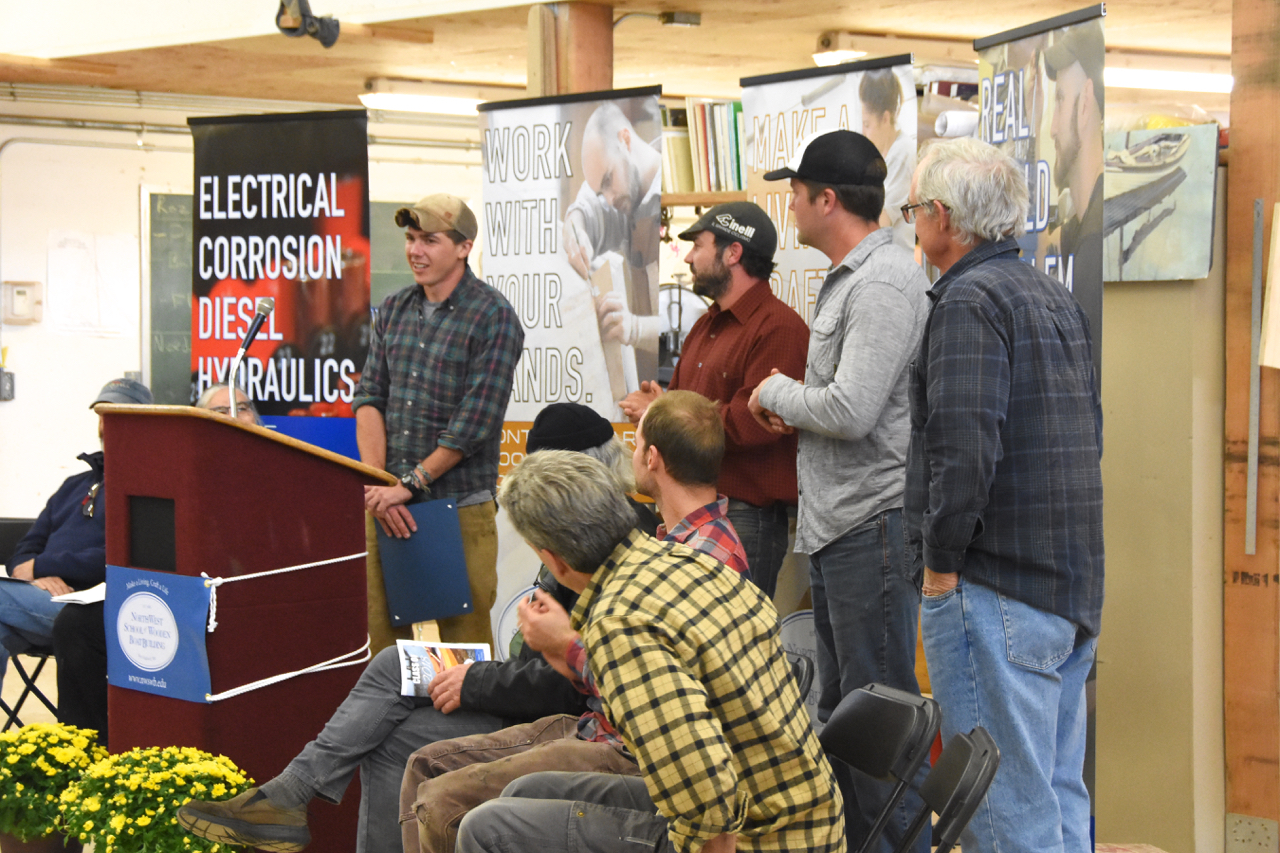This photograph depicts a group of men in a room, centered around a young man who appears to be giving a speech at a brown wooden podium equipped with a microphone. The young man, approximately 22 to 24 years old, stands confidently at the podium wearing a green baseball cap, greenish-colored pants, and a blue, red, and green plaid button-down shirt. He holds a navy blue folder or clipboard with four white dots in the corner, which might be a certificate. The room has cream-colored walls and a brown ceiling, and the setting is further adorned with yellow flowers placed in front of the podium.

Behind the young man, there is a series of banners with texts that read: "Electrical, Corrosion, Diesel, Hydraulics," "Work with your hands," and partially visible texts suggesting themes related to practical skills and career guidance. To his right, several men are either sitting in chairs or standing, watching him attentively. Specifically, three men are seated to the right side of the podium, with two men seated to the left, and three additional men standing behind those seated, all contributing to a sense of collective focus on the speaker. The overall scene suggests an educational or professional setting, perhaps a seminar, a class graduation, or a conference, highlighting vocational skills.